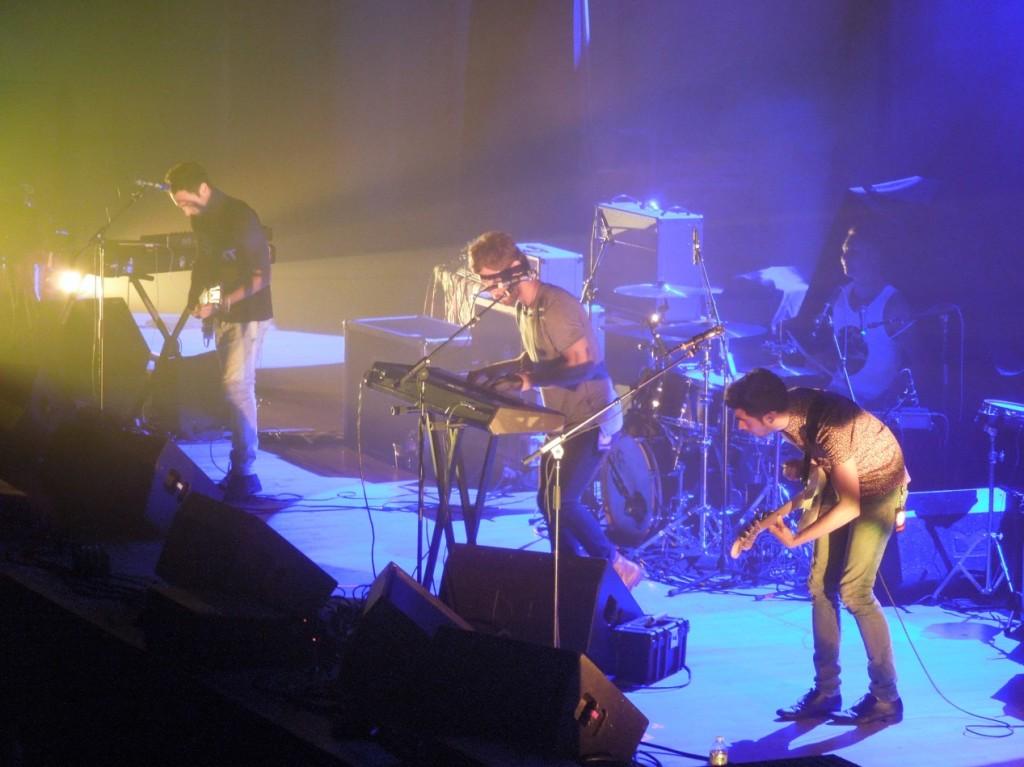This photograph captures a dynamic rock band in the midst of a live performance on a diagonally oriented stage, with the lower right leading towards the upper left. Three musicians are prominently positioned at the front of the stage: a crouching guitarist in jeans and a t-shirt is nearest the foreground, intensely focused on playing a riff. To his right is a keyboardist in a gray t-shirt and pants, captivating the middle of the stage. Further to the right is another guitarist in a dark t-shirt and jeans. Each of these front members has a microphone stand, although none appear to be singing at the moment. Behind them, partly obscured by the dim, blue-gray haze and smoke effects, is a drummer in a white tank top, working a large drum kit. The stage is bathed in spotlights, casting colorful highlights on the front musicians while the drummer remains cloaked in blue shadows. To the left and scattered around the scene are numerous amplifiers and speakers, with tangled cords visible on the floor. The environment suggests an electrifying atmosphere, punctuated by the vivid lighting and the musicians' vigorous postures, hinting at a high-energy performance in motion.